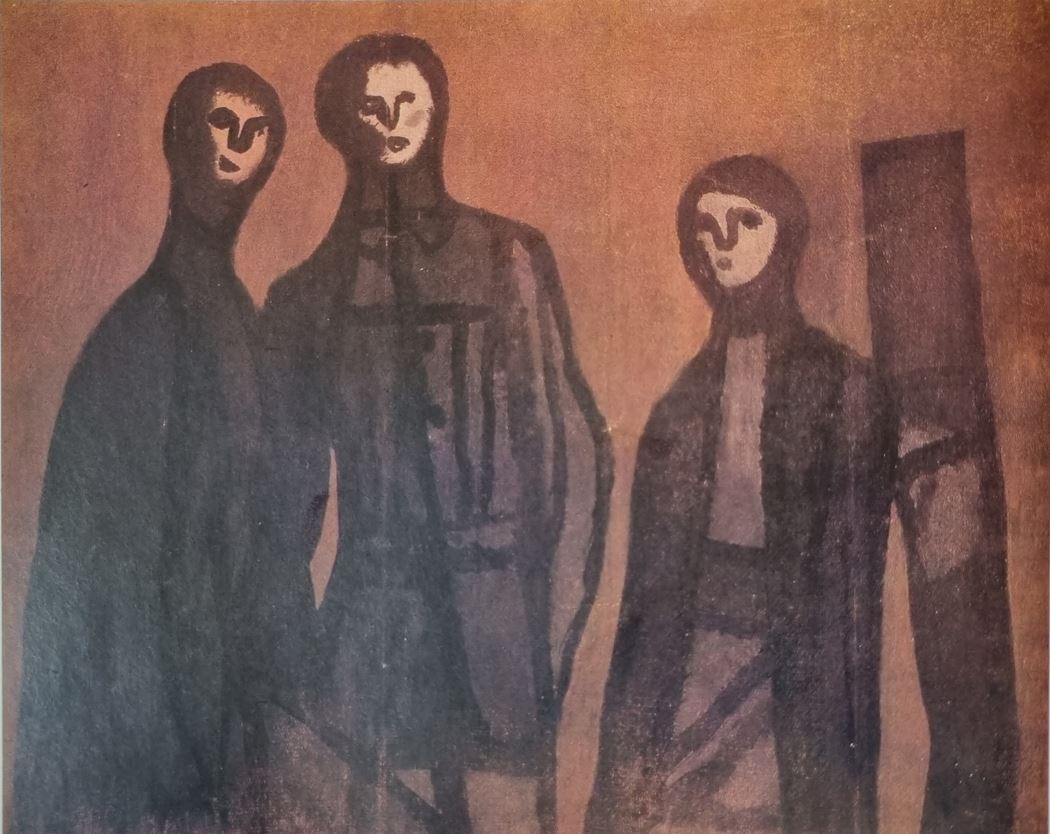This is a very expressionistic and modern drawing of three figures standing against a light brown backdrop. Each figure has a white face with rudimentary features: small black circles for eyes, a simple line down the face forming a nose, and tiny black dots for mouths. The figures are dressed in black suits with dark jackets, one of which appears partially see-through, revealing seams and dark buttons. The tallest figure in the center wears a jacket with buttons, giving an impression of a uniform. The figure on the right is leaning against what could be a post or a door, and their jacket appears to be partially open with a dark-colored waistband. The style is very contemporary and two-dimensional, with a flat, monotone color scheme dominated by blacks, grays, and some light brown for the background. The simplicity and lack of detailed features lend a mysterious and unusual quality to the artwork.